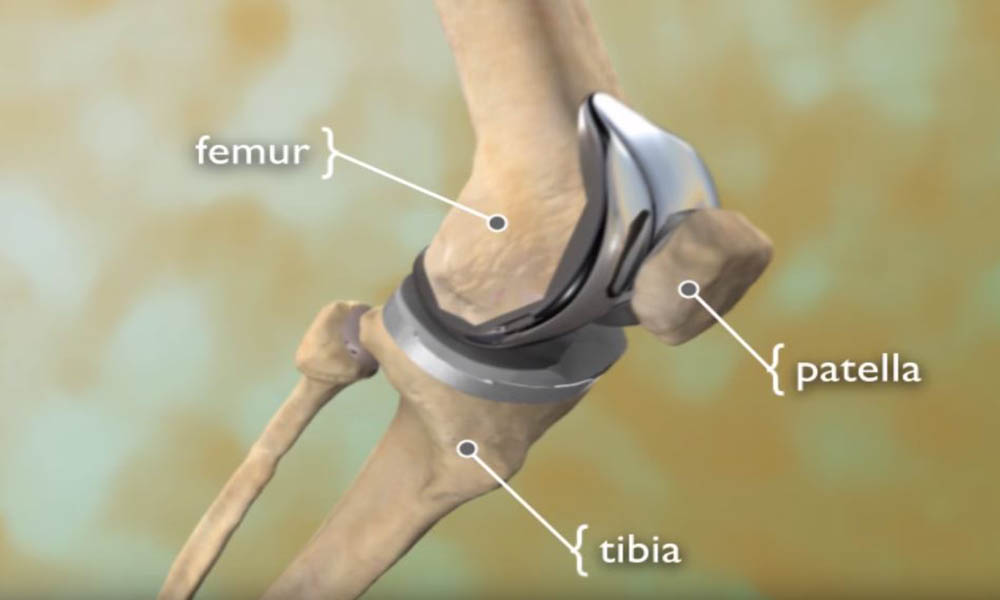The image is a rectangular, close-up view of an artificial knee joint, featuring detailed labels and a muted, blurred background in shades of greenish-gray and beige. The main focus is on three beige-colored bones: the femur at the top, the patella or knee bone in the middle, and the tibia below it. Each bone has a white label with corresponding white arrows: "femur" for the top bone, "patella" for the middle bone, and "tibia" for the bottom bone. Between the bones, particularly between the femur and tibia, there are silver metal components, indicative of an artificial knee replacement, likely representing medical prosthetics used to replace worn-out tendons or ligaments. The setup suggests the image is part of a medical diagram, possibly something a doctor would use for explanation or educational purposes.